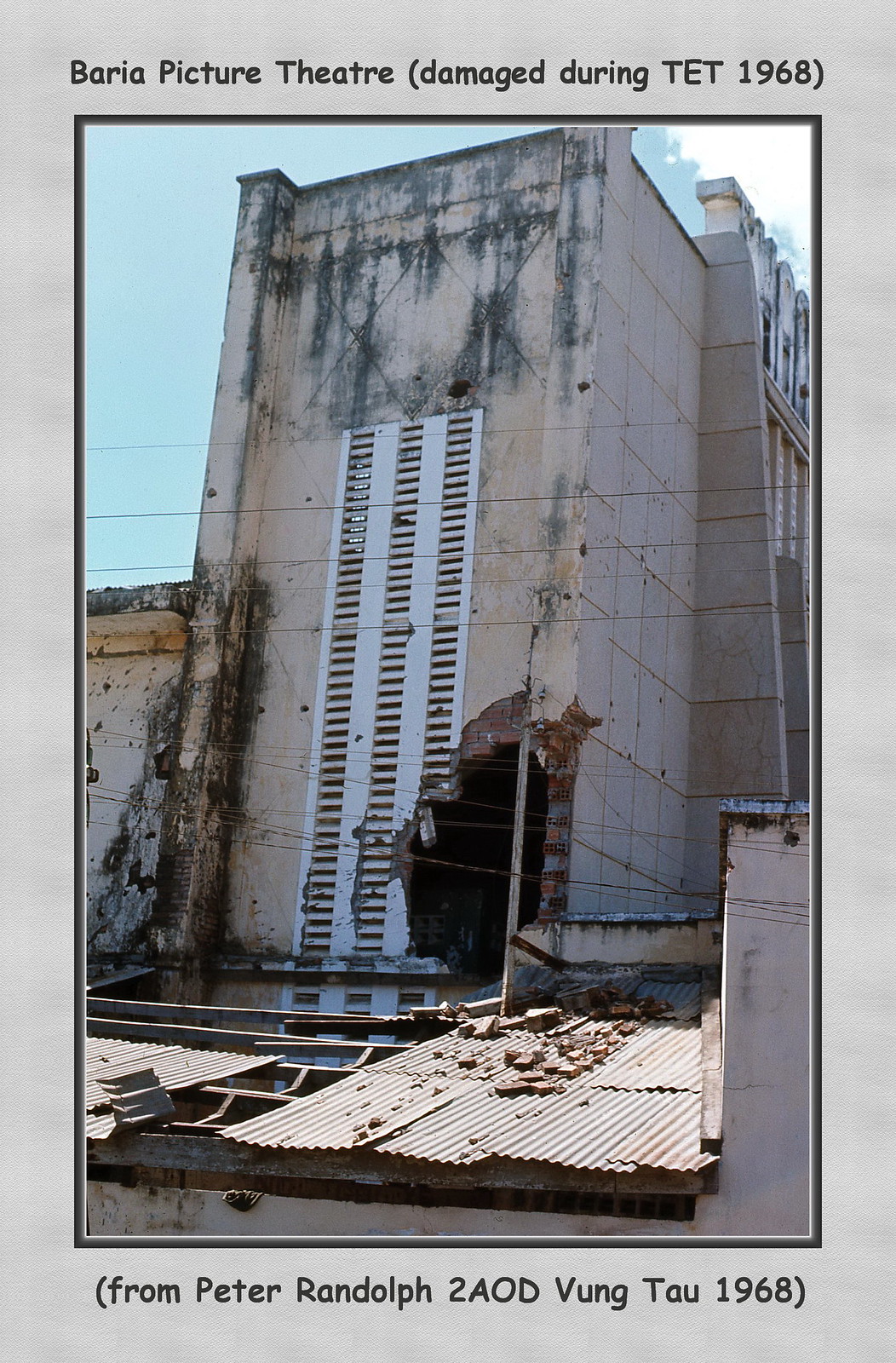The image depicts the heavily damaged Barrier Picture Theater during the T.E.T. Offensive of 1968, as indicated by the title at the top and the photographer's note at the bottom which reads, "from Peter Randolph to A.O.D. Vung Tau 1968." The theater appears to have sustained considerable damage, with a large hole prominently visible in the bottom right corner, likely from a bombing. The structure shows significant wear, with a stained or moldy appearance at the top, and what seems to be a missing door. The left pillar and other parts of the building are clearly damaged. The ground is littered with debris, including pieces of the wall or possibly a fence, along with wood and bricks. Despite the destruction, the scene is set in broad daylight with no individuals present, highlighting the desolation. The photo is framed in a digital format and starkly captures the aftermath of the violence inflicted upon the once-standing theater.